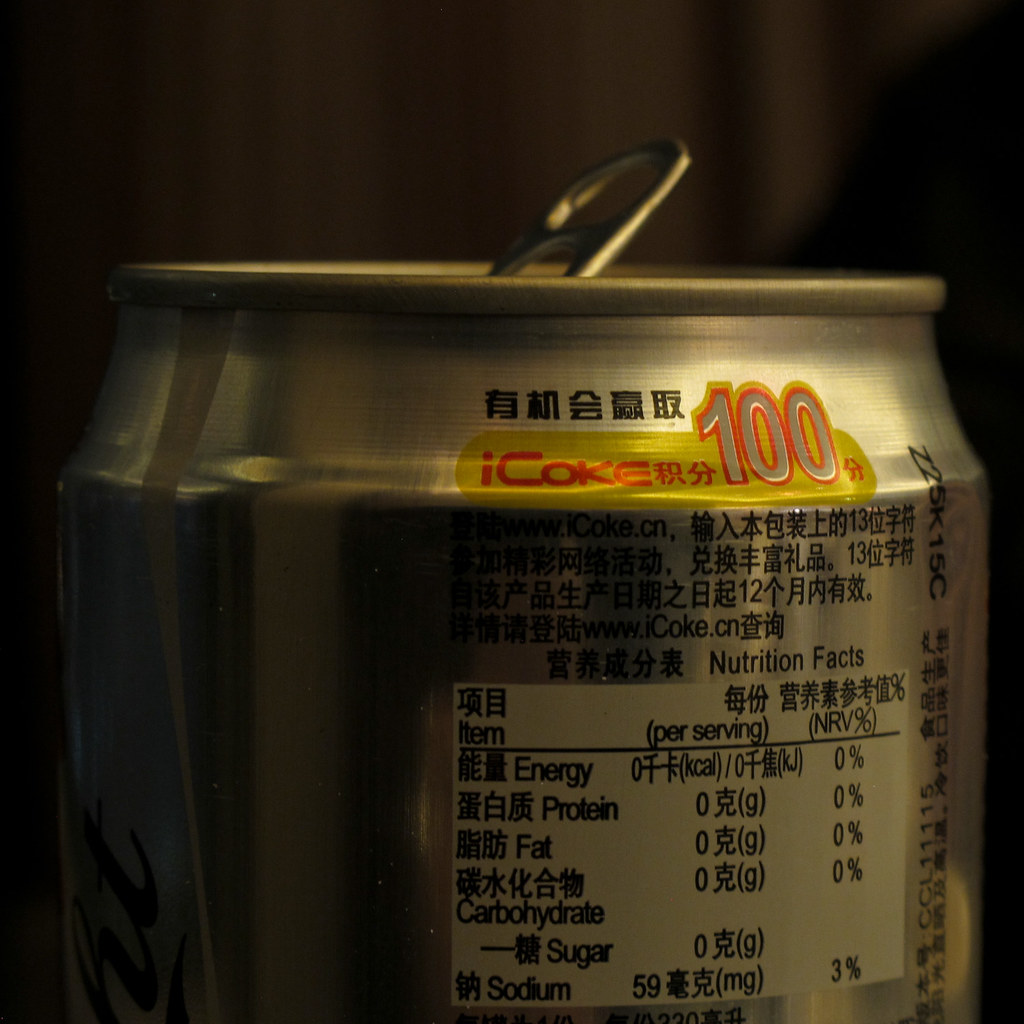This image is a detailed, close-up shot of a silver Coca-Cola can, specifically the I-Coke variant, marketed in a Chinese-speaking region as indicated by the language on the can. The foreground features the metallic sheen of the aluminum can, prominently displaying the partially lifted pull tab at the top, suggesting the can has been opened. The setting appears fairly dim, with a dark background that makes the can's textures and details stand out, accentuated by subtle lighting that casts a shadow over the top.

Prominently visible below the pull tab is a horizontal promotional banner in a yellow background with red text stating "I-Coke 100", indicating a promotional campaign likely offering prizes or rewards. The text above and below this banner is predominantly in Chinese, although there are some English words present such as "nutrition facts," "energy," "protein," "fat," "carbohydrate," "sugar," and "sodium per serving," along with an NRV percent figure. Additionally, there is an English web address "www.icoke.cn," confirming the can's marketing in a Chinese-speaking region. The overall combination of metallic silver with red, white, and black graphics makes for an eye-catching design against the dark backdrop, emphasizing the can's sleek, modern appearance.